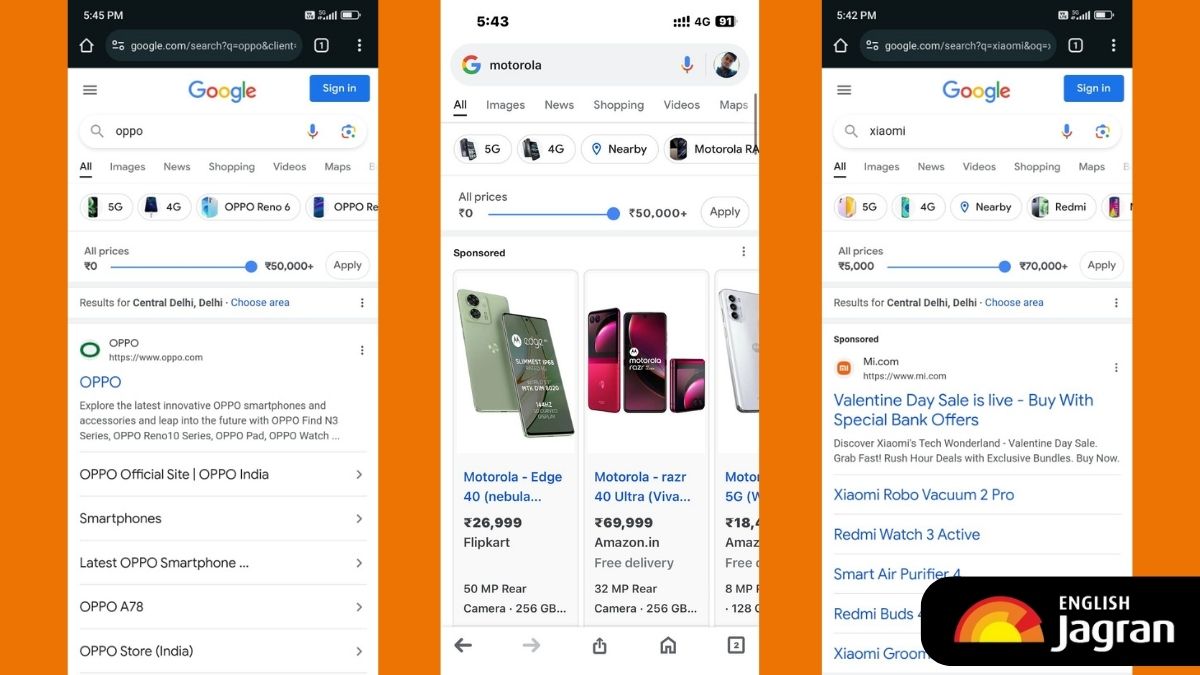The image is a composite screenshot showcasing three different mobile webpage searches, each for a different smartphone brand. At the bottom right corner, there's an icon labeled "English Degran" accompanied by a red and yellow symbol. 

The first screenshot displays a search for "Oppo," with results specifically from Central Delhi, Delhi. The display highlights the Oppo website, suggesting that Oppo is a company specializing in smartphones and other technology devices.

In the second screenshot, the search query is "Motorola." The status bar shows the time as 5:43, a 4G cellular indicator, and the battery percentage. An adjustable price range filter is visible, spanning from 0 to over 50,000. The top portion of the search results features a sponsored section with various advertised Motorola smartphones.

The third screenshot captures a search for "Xiaomi," with prices ranging from 5,000 to 70,000. Similar to the first search, the results are from Central Delhi, Delhi. The page includes a sponsored section for me.com, promoting a Valentine's Day sale with special bank offers, and presents a list of clickable products available for purchase.